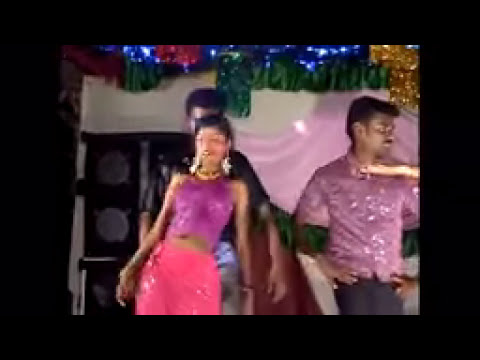The image depicts a bustling dance event, likely inspired by Tamil Nadu traditions, hosted in a vibrantly decorated dance pavilion. Streamers and glittering gold decorations hang from the ceiling, casting a festive atmosphere reminiscent of a grand celebration. In the background, a wall adorned with decorations similar to those used during New Year's Eve celebrations showcases a stack of black rectangular speakers with prominent circular elements. Despite the overall blurriness, three main figures stand out: a woman with long, exotic earrings is in mid-dance, wearing a sparkling sleeveless top that appears purple and a pink, gold-highlighted skirt. Beside her, a man with a shimmering pink shirt and black pants stands with his hands on his hips, looking off to the side, seemingly engaged in a conversation. Another man is partially seen in the background, seemingly on the move. The vivid colors and sparkling outfits of the dancers, combined with the elaborate decorations, suggest an exuberant celebration of Indian cultural dance from Tamil Nadu.